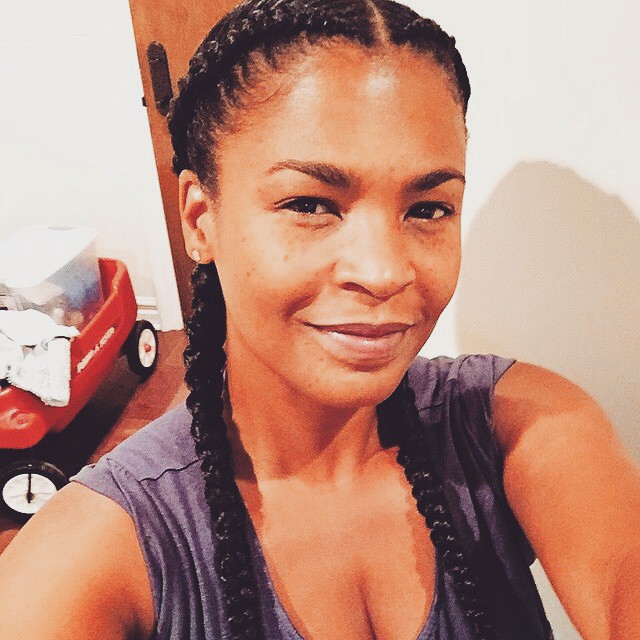The image showcases a young African descent woman, Nina Long, taking a selfie. She is wearing a gray short-sleeved t-shirt, which she appears to have tucked the sleeves inside, revealing a touch of cleavage. Her hair is styled in two long braids that fall across her chest, and she sports dark brown eyes, a smattering of freckles across her face, and a small stud earring. She is slightly smiling with her mouth closed, and her well-groomed eyebrows accentuate her natural look. The background features a red plastic toy wagon with a plastic bin containing some items, possibly including a white coat, adding to the impression of a cluttered indoor setting. The setting is further complemented by white walls and a brown wooden door, suggesting the photo was taken inside her home.